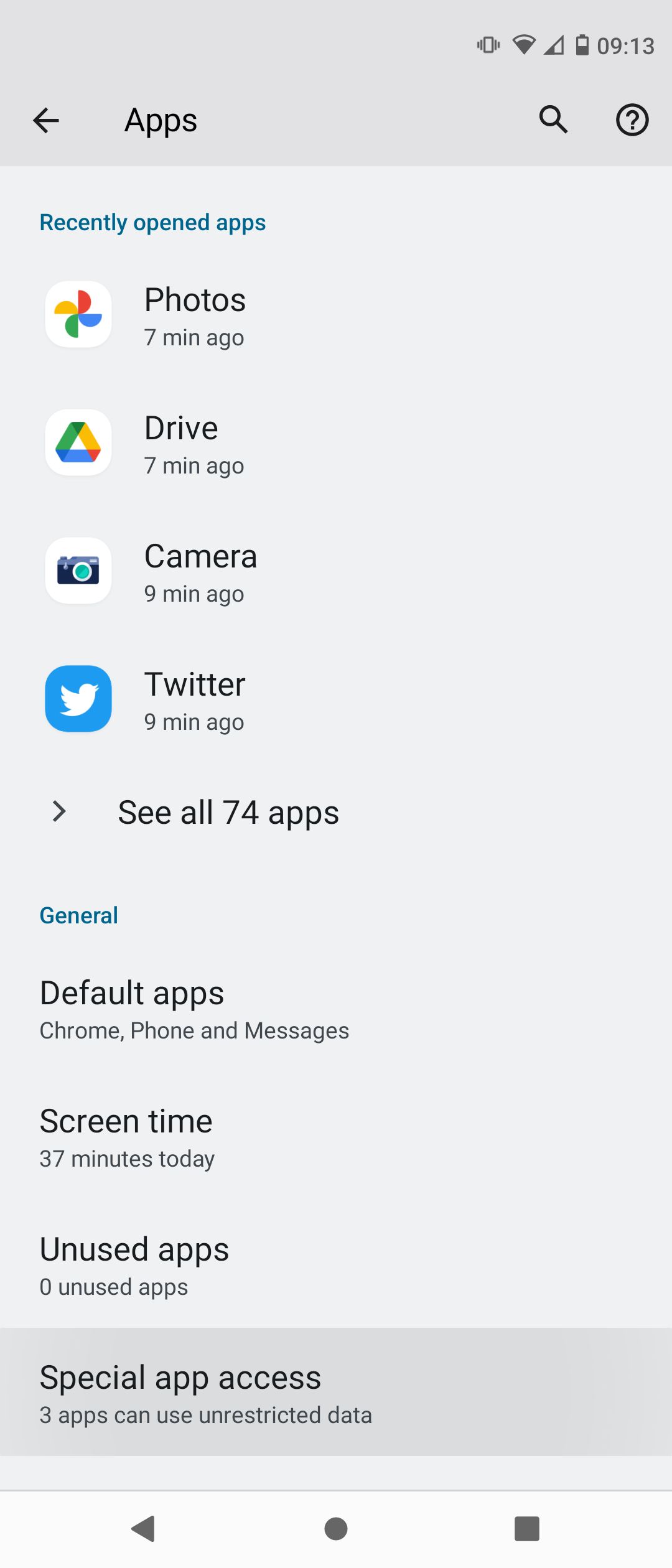In this detailed screenshot, captured from a smartphone, we see various status icons located at the top left corner of the screen: a vibrate icon, Wi-Fi icon, network signal icon, battery icon, and the current time displayed as 9:13. The background color of the screen is light gray.

In the interface, the page title prominently reads "Apps" at the top, with a search icon to the right followed by a help icon. Below the page title, there is a section labeled "Recently opened apps" in blue text. The listed apps, named in black text, include:

1. **Photos** - Opened seven minutes ago, represented by an icon featuring a white background with a combination of red, green, yellow, and blue colors.
2. **Drive** - Also opened seven minutes ago, marked by a triangle icon with the same colors as the Photos app.
3. **Camera** - Opened nine minutes ago, displayed with a camera icon.
4. **Twitter** - Opened nine minutes ago, indicated by a bird icon in white set against a blue background.

At the end of this section, there is a link in blue that reads "See all 74 apps."

Further down, a section labeled "General" (in blue text) provides the following information in black text:
- **Default apps:** Chrome, Phone, and Messages.
- **Screen time:** 37 minutes a day.
- **Unused apps:** Zero unused apps.
- **Special app access:** Three apps can use unrestricted data.

The active selection, "Date," is highlighted in a slightly darker gray than the background color.

At the very bottom of the screen, there are three navigational buttons for the smartphone: a square, a circle, and a triangle, used for different standard actions.